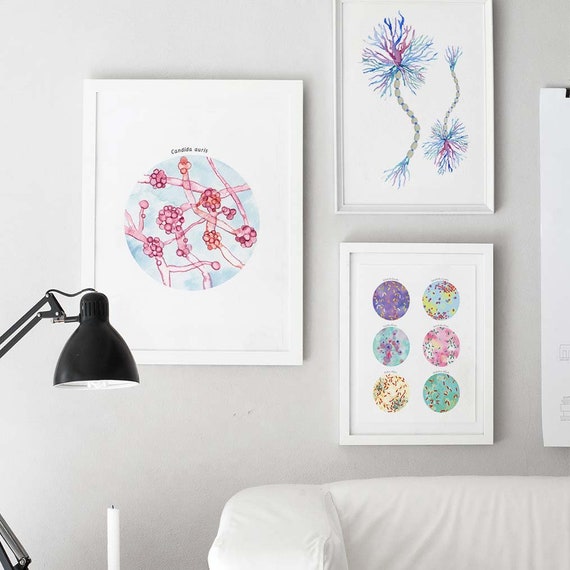This is a detailed photograph of a living room taken from an angle that captures a part of the front wall and the right side of the room. The front wall, painted off-white, features three white photo frames, each showcasing colorful drawings that appear to depict organisms and microscopic images. These pieces of art add a splash of color to the otherwise muted room. On the left side of the image, a black table lamp with its head pointing downwards is visible, suggesting it sits atop an end table which is cropped out of the photograph. At the bottom right corner, part of a white couch is seen, with its backrest included in the frame while the bottom part is cropped out. The overall shape of the photograph is square, capturing an intimate and somewhat abstract glimpse into a cozy, yet artistically decorated living space.